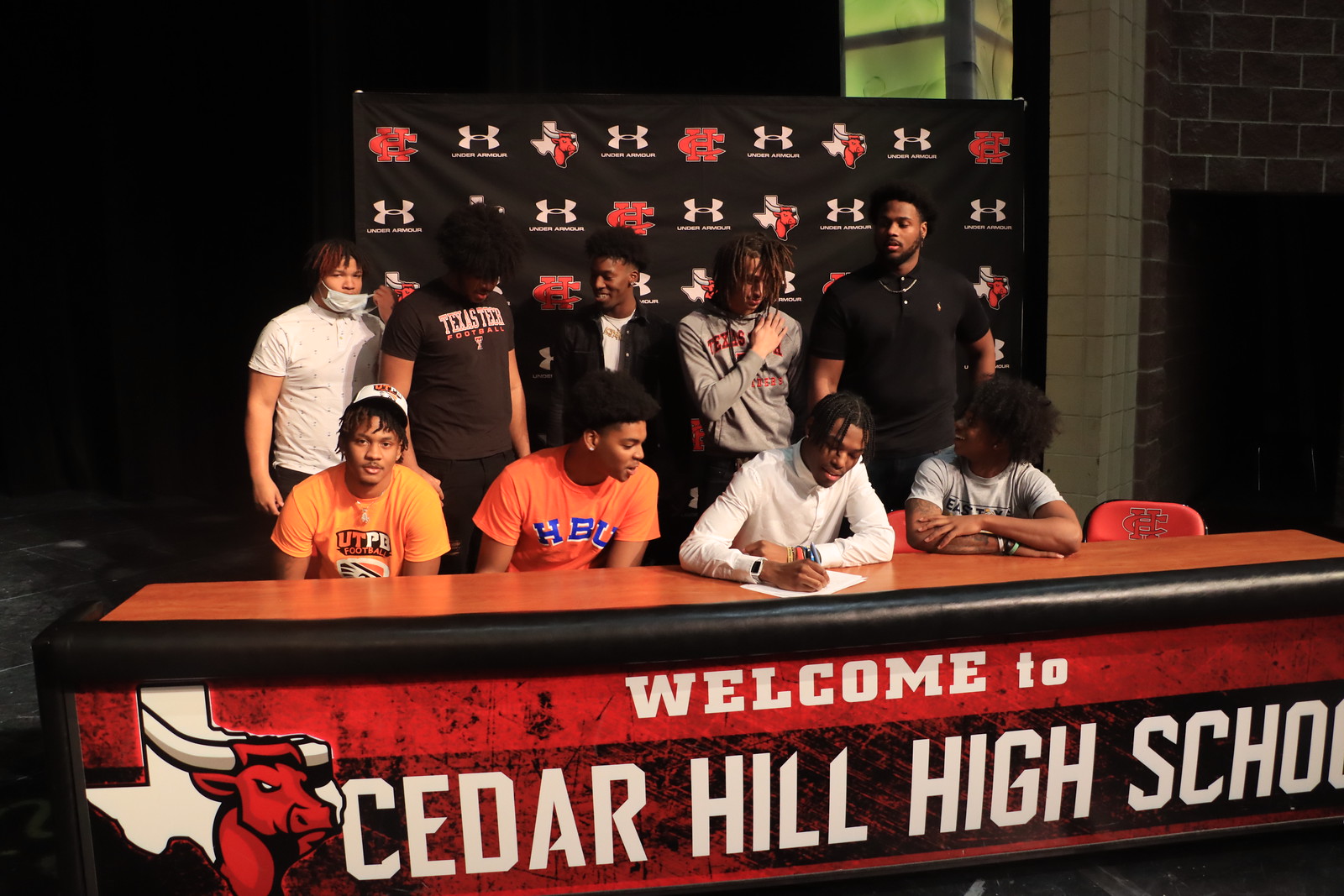In an indoor photograph taken in a dimly lit room, a long, narrow wooden table with black-cushioned edges stretches from the bottom left corner slightly upward to the right. Draped across the front of the table hangs a red banner with white text that reads, "Welcome to Cedar Hill High School," accompanied by a white outline of the state of Texas with a red longhorn inside on its left side. Seated at the table are four men of African descent, surrounded by five men standing behind them, four of whom are also of African descent, with one appearing to be Caucasian. A backdrop behind them features a black background patterned with repeated sponsor logos, including a red letter 'C' intertwined with a red letter 'H,' the Under Armour logo, and the white state of Texas with a red longhorn. To the right, the room reveals red brick walls and a white brick column at the corner where the wall curves, suggesting a setting prepared for an official event, possibly related to basketball tryouts or recruitment.